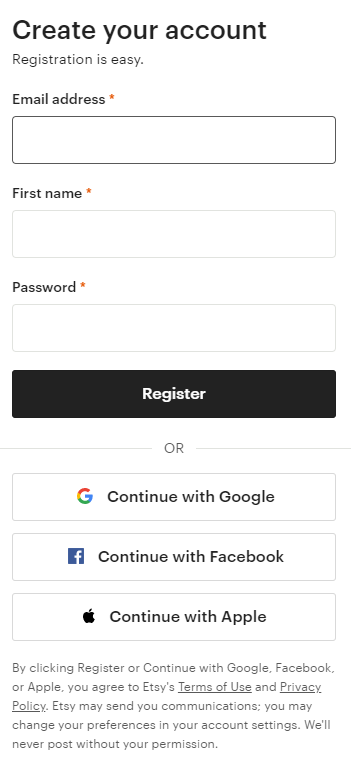This image depicts a "Create Your Account" registration page for signing up on a website. The heading "Create Your Account" is prominently displayed in large, bold, black font, and is left-justified at the top of the form. Beneath this heading, the subtext "Registration is easy" is aligned to the left and written in a smaller font.

Following this, a space separates the subtext from a series of form fields and labels. "Email Address" is written in bold, with a small red asterisk indicating it’s a required field. Directly below this label is a text input box for entering an email address. Another space follows before the next section labeled "First Name," also bold with a red asterisk. Below this label is a text input box to enter the first name.

A similar pattern continues for the "Password" field, which is bold with a red asterisk to indicate it’s required, and a corresponding text input box below it.

Below these input fields, another space is followed by a "Register" button. Underneath the button, the word "or" is placed to provide alternative registration options. These alternatives are: "Continue with Google," "Continue with Facebook," and "Continue with Apple," giving users the flexibility to sign up using these services.